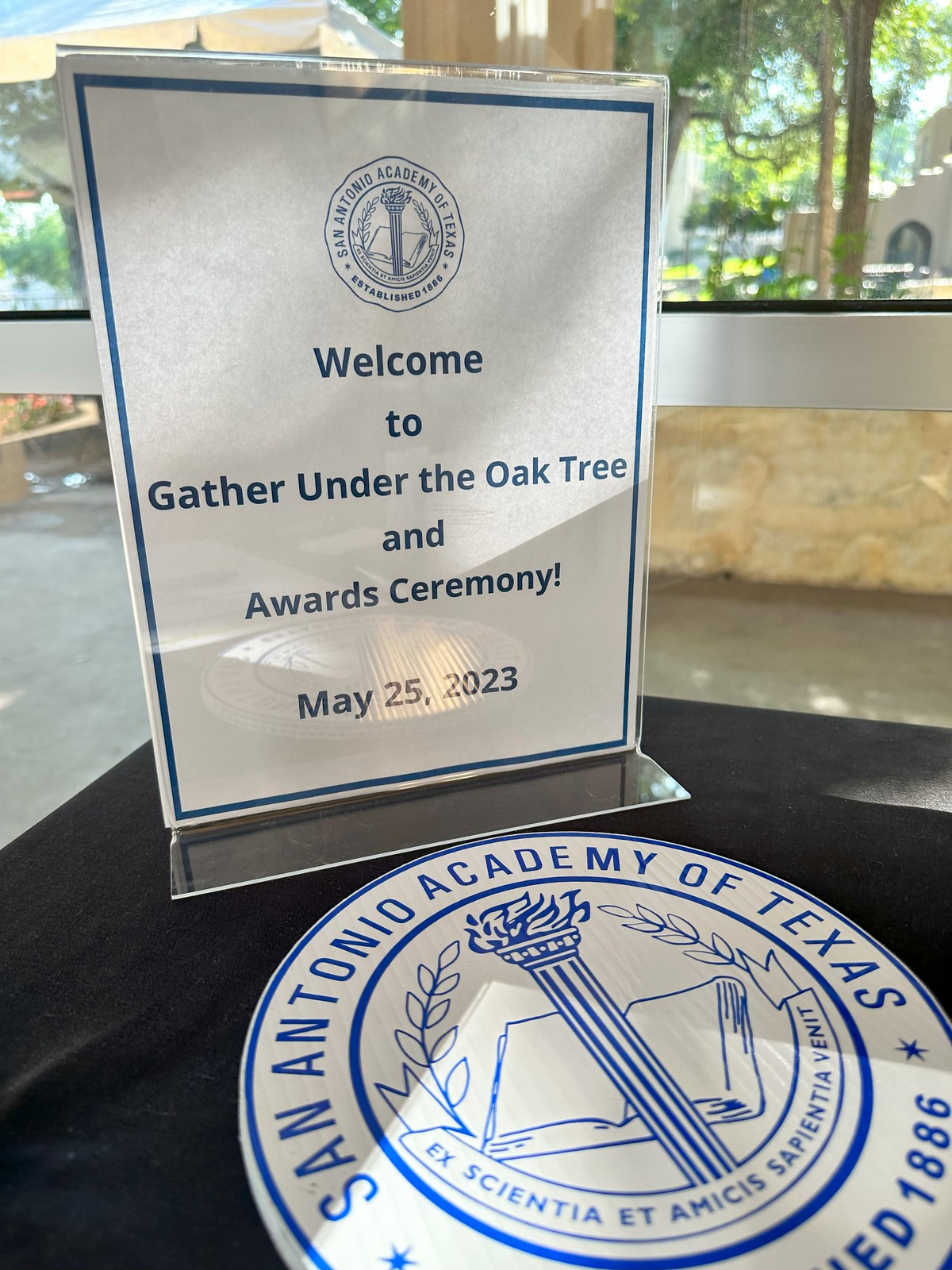The image depicts a white paper sign encased in a clear plexiglass holder with small feet. The sign, placed on a black table, prominently displays a blue insignia at the top center which reads "San Antonio Academy of Texas, Established 1886." The insignia features a central column topped by a torch, flanked by fig leaves reminiscent of Olympic iconography, and has the Latin phrase “Ex Scientia et Amicus Sapientia Evente” inscribed at the base. The text on the paper sign announces, "Welcome to Gather Under the Oak Tree and Awards Ceremony, May 25th, 2023." Behind the sign, there are large windows revealing a garden area with trees and greenery, suggesting an elegant event setting.